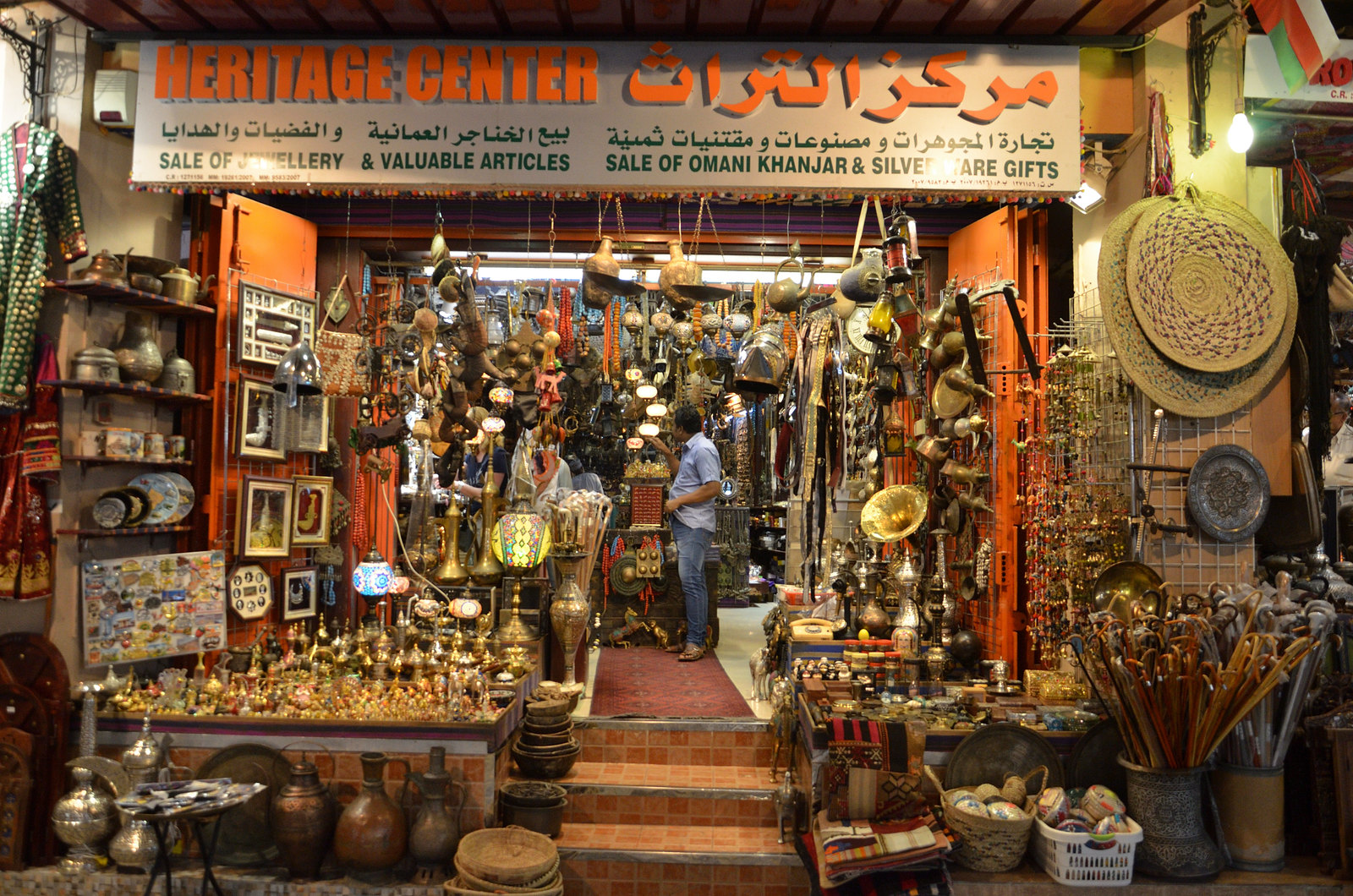The image showcases the bustling front of the "Heritage Center" shop, marked by a gray marquee with red text declaring its name, and additional text in green and English detailing the sale of jewelry, valuable articles, Omani Kanjar, and silverware gifts. The store is brimming with a myriad of colorful items, creating a crowded, bazaar-like atmosphere. On the left, a bucket of multicolored canes stands out, alongside piles of baskets, large woven mats, plates, and urns made of clay, copper, and silver. Gold trinkets and large brown vases gleam among the assortment of utensils, pots, pans, and various hanging items adorning the walls. There's a clear pathway with orange tiles and a red carpet leading into the store. A man, dressed in a blue shirt and jeans, stands in the center, partially turned toward the camera, adding a human element to this vibrant and eclectic scene.